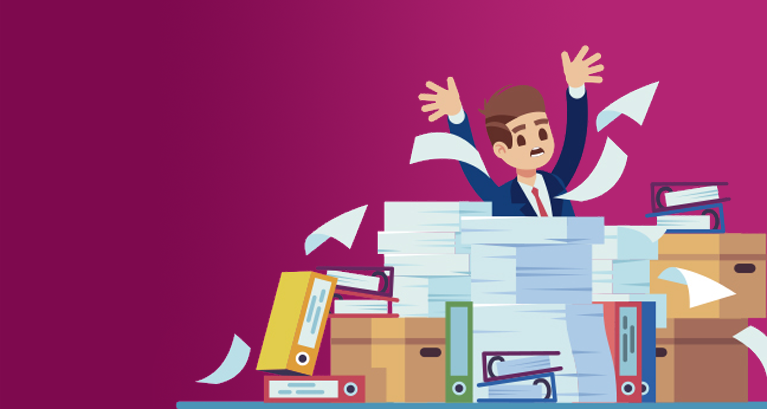This cartoon image depicts an office worker, clad in a blue suit, white shirt, and red tie, in a state of visible stress and frustration. The character, with short brown hair, expressive cartoon eyes, and an open mouth, has his hands thrown up in the air, fingers spread wide. Surrounding him are three towering stacks of white paper, three file boxes, and an assortment of binders—some arranged vertically wedged between the boxes and paper stacks, while others are scattered on top of the file boxes. The binders are vividly colored in red, blue, green, and yellow. Papers are seen flying and falling around him, indicating a moment of chaos. Shadows cast by the stacks and boxes add depth to the scene. The background transitions from a darker to a lighter purple, enhancing the chaotic atmosphere, reminiscent of something seen on a website homepage.